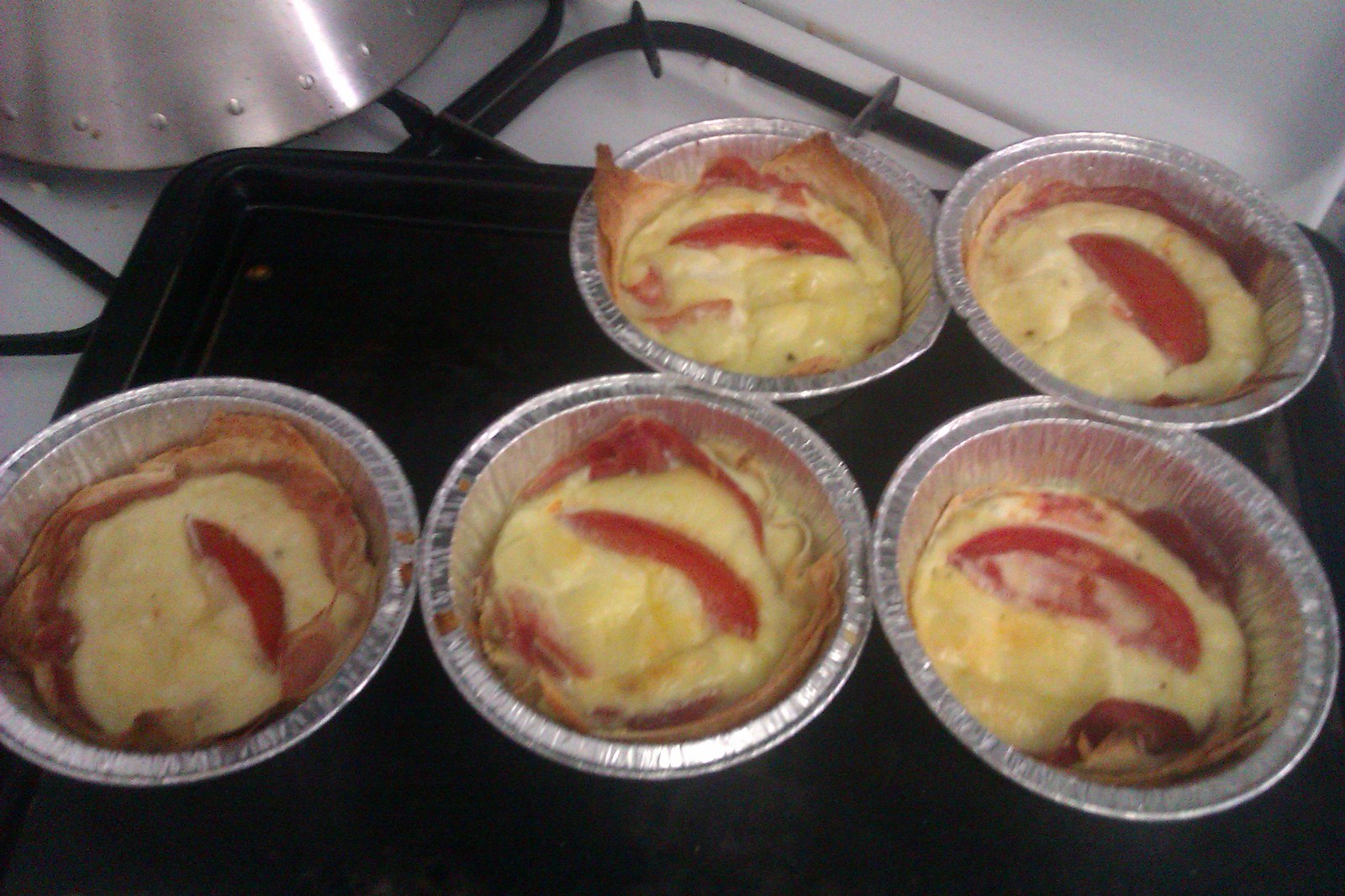The image shows five small, circular aluminum pie tins arranged on a black baking sheet. Each tin appears to be filled with puff pastry as the base layer, topped with a layer of melted white cheese, and garnished with a slice of tomato. The tins are shallow, with some corners of the puff pastry or tortilla poking out. The setup is placed on a white gas stove with black grates. In the top left corner of the image, a silver kettle or coffee pot is partially visible. The photo quality suggests it was taken with a phone.